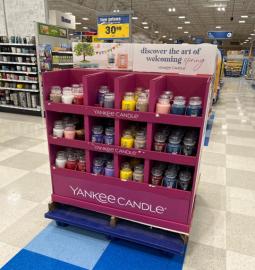This is a detailed photograph of a well-lit craft or hobby store featuring a central Yankee Candle display. The main attraction of the image is an end cap display constructed from a fuchsia-colored cardboard or similar material. The display consists of 12 open compartments arranged in three rows of four. Each compartment is filled with various Yankee Candle jar assortments showcasing a vibrant array of colors, including pink, yellow, green, dark blue, red, brown, white, and purple. Above the display, a sign reads "Discover the Art of Welcoming Spring," accompanied by an image of a tree and jars of candles. The display rests on a blue mat, which is surrounded by alternating light gray and white tiles in a checkerboard pattern. The background reveals additional shelves and displays, though the details of their contents are blurry. Illuminated price signage, presumably indicating $30.99, is visible, suggesting a possible Walmart location known for its characteristic blue and yellow color scheme. The large, well-polished floor space and high shelving unit indicate this is within a significant retail store setting.